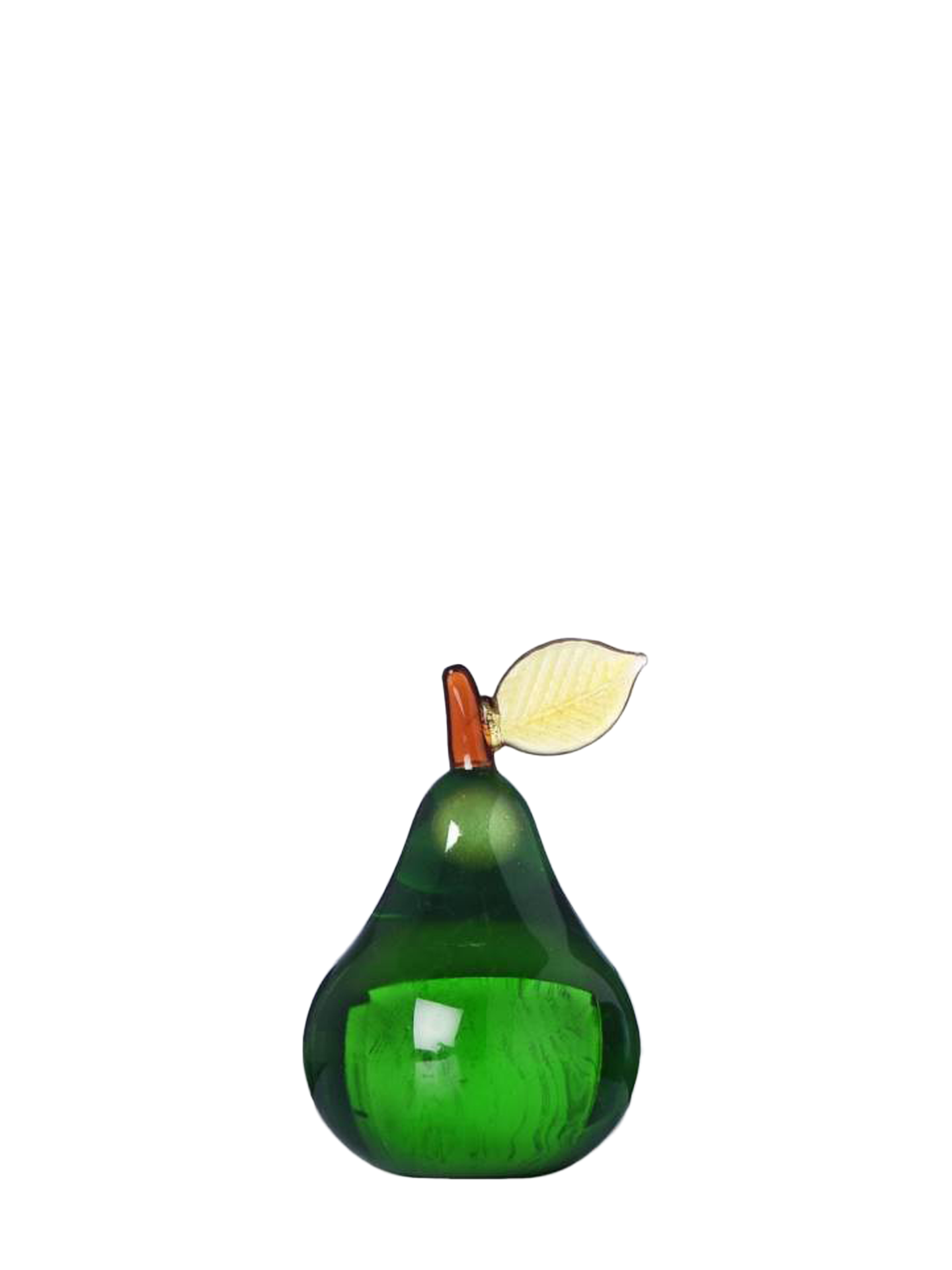The image features an intricately designed glass canister shaped like a pear, characterized by its glassy green body that transitions from a darker hue at the base to a lighter, almost white tint in the middle and top portions. The pear shape is emphasized by its wider base and narrowing top, crowned with a brown, glassy stem. At the very top, a translucent, yellow glass leaf with detailed ridges is attached to the stem, adding a touch of realism to the artistic piece. Inside the canister, the green glass exhibits varying shades and textures, suggesting there may be an object like a candle within, although it is not clearly visible. The image is focused solely on the glass pear, with no contextual background elements.